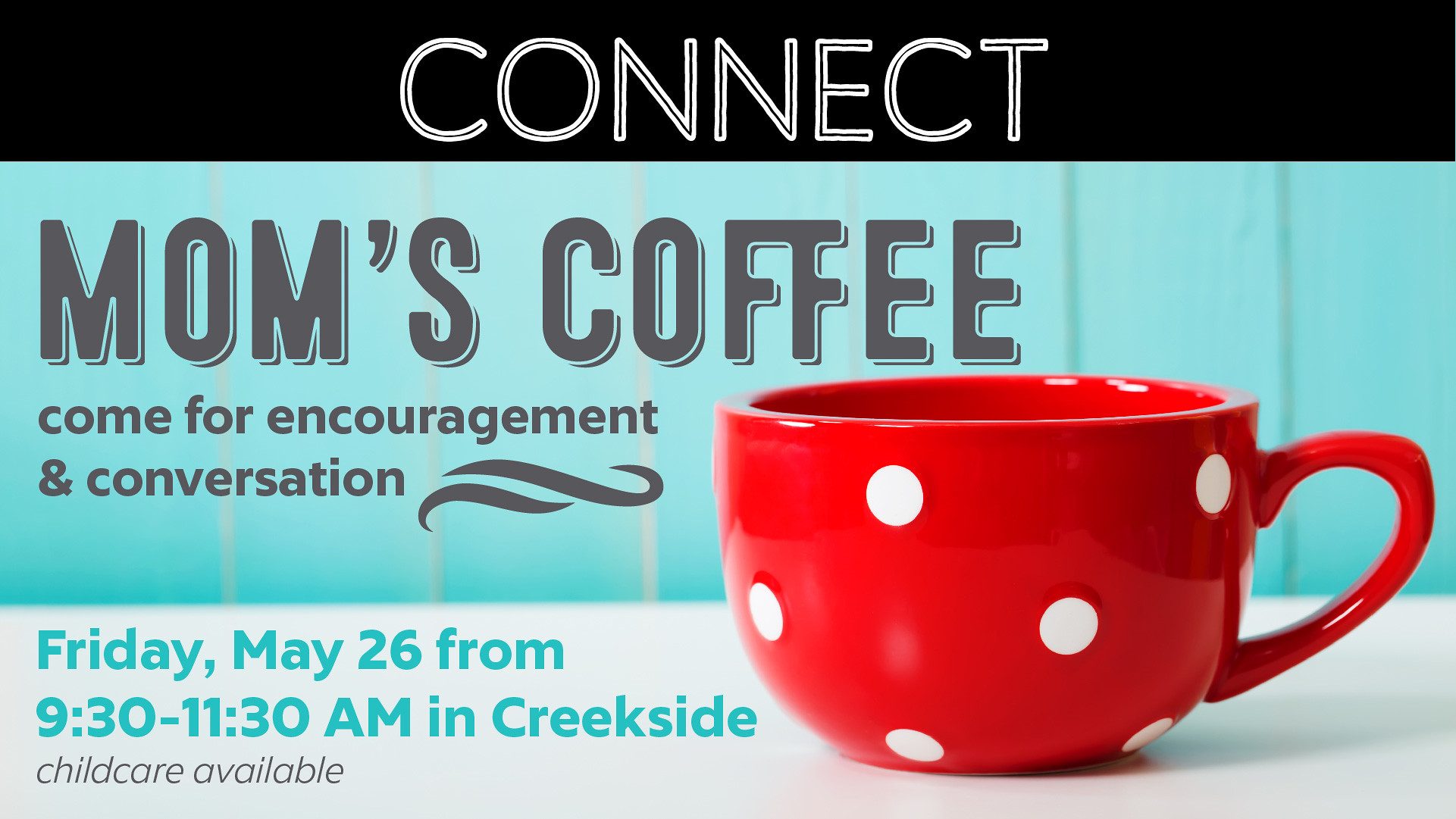This image is a wide rectangular advertisement for an event, styled similarly to the dimensions of a high-definition TV. Dominating the top portion is a thick black rectangle, spanning the width of the image. Centered within this rectangle, thin white capital letters spell out "CONNECT," separated by a thin black line. Below this, the right side of the advertisement features a vivid photograph of a shiny red coffee cup adorned with white polka dots, positioned with its handle to the right. The cup rests on a pristine white surface.

The backdrop behind the cup appears slightly blurred and consists of vertically arranged light blue wooden planks. To the top left of the coffee cup, in dark gray font encased within a light blue border, the text proudly announces "MOM'S COFFEE." Beneath this, in matching dark gray letters, the invitation continues with "COME FOR ENCOURAGEMENT AND CONVERSATION." Further down, in clear turquoise font, the details of the event are specified: "FRIDAY, MAY 26TH FROM 9:30 TO 11:30 AM IN CREEKSIDE." Finally, at the bottom of the text, it reassures attendees with the phrase "Child care available." The image likely combines a photographic element with text overlays added through digital editing software like Photoshop.